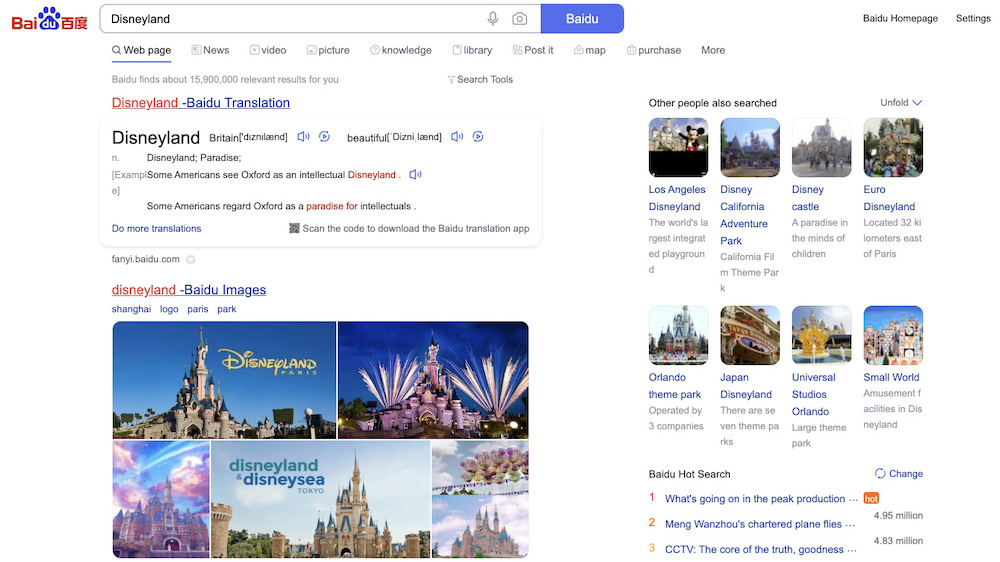In this image, a user appears to be searching for "Disneyland" on the Baidu search engine, as evidenced by the search bar at the top. The Baidu interface features a selection menu with options such as Web Page, News, Video, Picture, Knowledge, Library, Post-it, Map, Purchase, and More, with "Web Page" being currently selected. Below the search bar, the top search result reads, "Some Americans see Oxford as an intellectual Disneyland."

Further down, there is an image section titled "Disneyland Baidu images," showcasing various pictures. The first row features a prominent picture of Disneyland's iconic castle surrounded by fireworks. Subsequent images include the Disneyland castle, Disneyland in DisneySea, and repeated castle images. 

On the right side of the screen, there are additional search suggestions under "Other people also searched," listing connections to Los Angeles Disneyland, Disney California Adventure Park, Disney Castle, Euro Disney, Orlando Theme Park, Japan Disneyland, Universal Studios Orlando, and Small World. 

Finally, at the bottom right corner, there is a "Baidu hot search" section with current trending topics, mentioning "what's going on in the peak production" and "Ming Wenzhou's character playing flies."